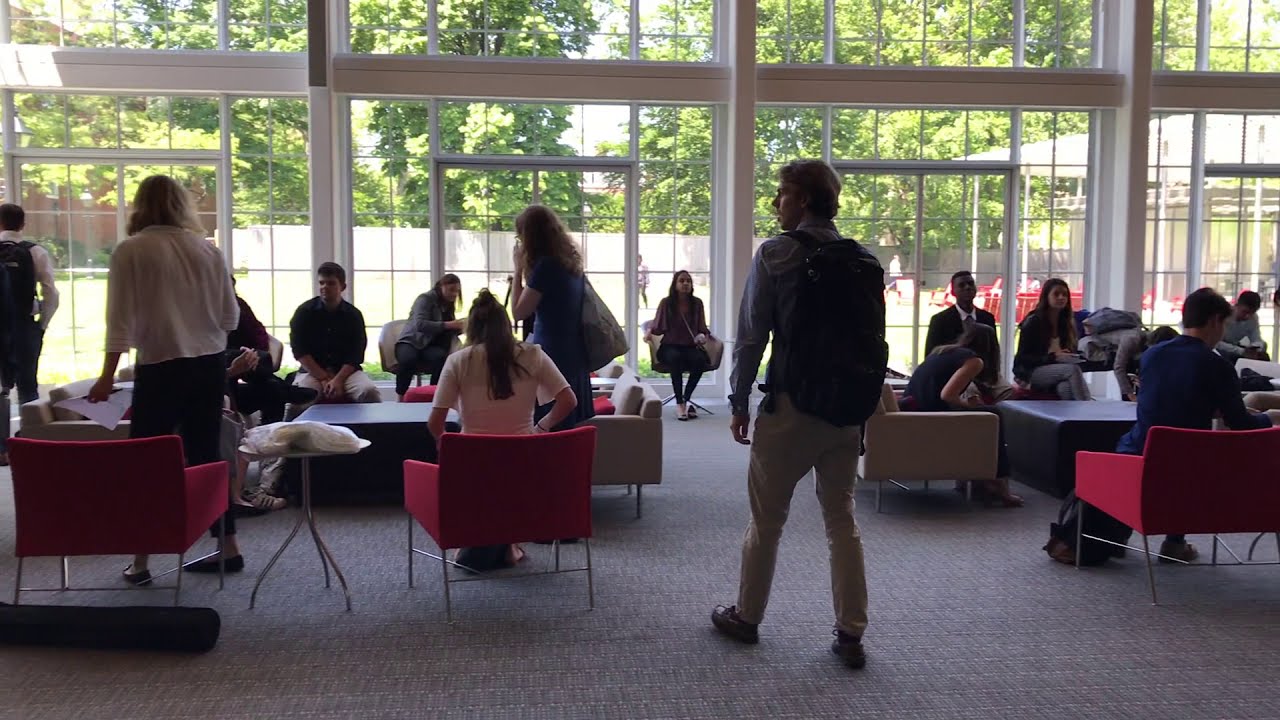This detailed color photograph is a horizontally aligned rectangular image capturing a lounge area inside a large, open room, potentially on a college campus or an office building. The floor is covered with a very thin, subtly patterned brownish-gray carpet. The room is furnished with a mix of low red and gray padded chairs and small black tables.

Central to the image is a man with short brown hair, wearing khaki pants, a long-sleeve shirt, and a black backpack. His back is mostly to the viewer, slightly turned to the side. Scattered around him are people in their twenties, sitting or standing, some holding bags, creating a relaxed, social atmosphere.

The background of the room features a wall composed almost entirely of large square windows, which provide a clear view outside. Visible through these windows are a gray stone wall, a sidewalk, tall trees with green leaves, and other outdoor elements like a fence and a small pagoda, all illuminated by natural sunlight streaming into the room. The overall scene suggests a bright and sunny day, contributing to the casual, open feel of the lounge space.